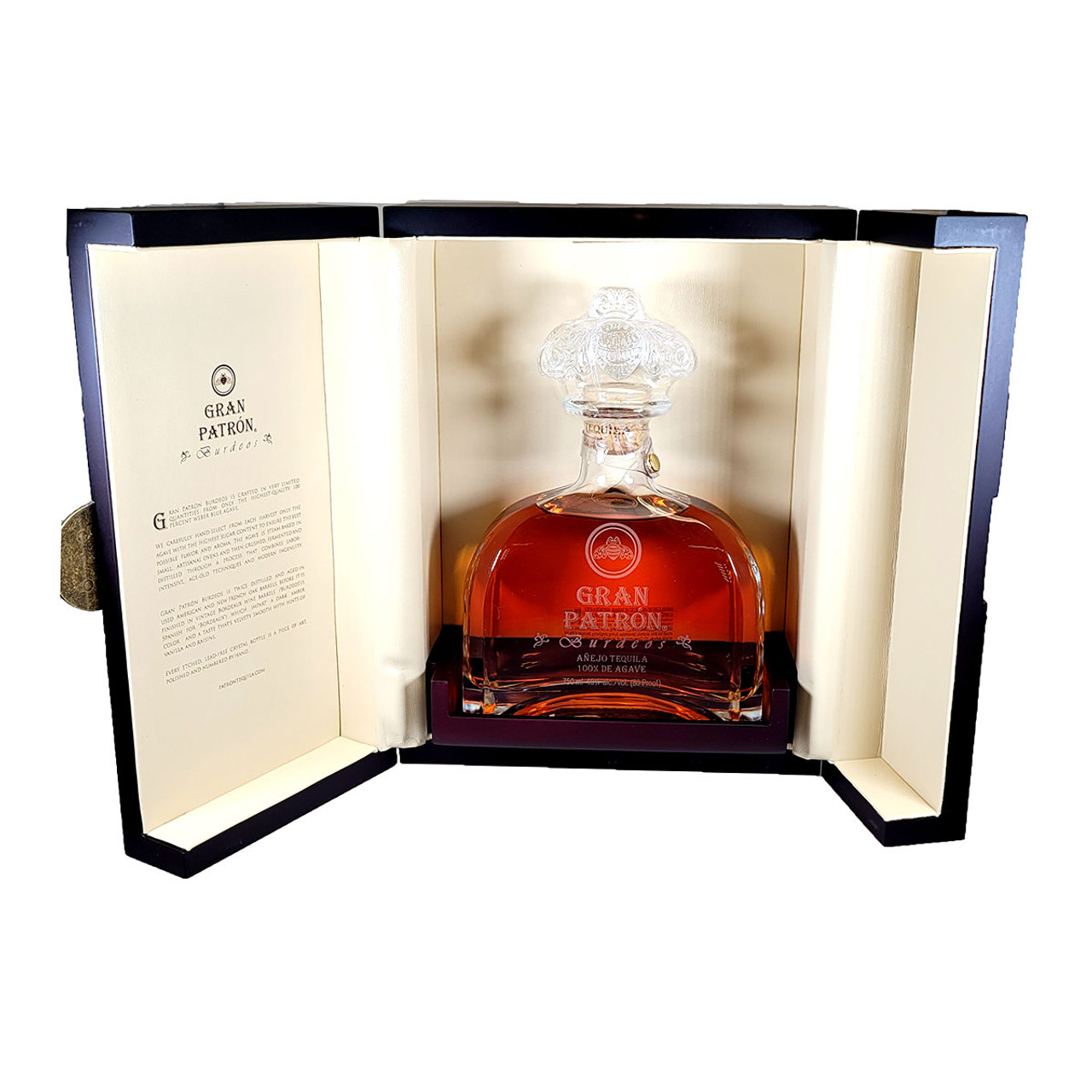The image features a bottle of Grand Patron Barracos Anejo Tequila, exquisitely showcased in a sophisticated gift box. The box's interior is primarily beige with a black rim, and contains multiple paragraphs of text likely detailing the tequila's origin, production process, and other pertinent information, although the text is too blurry to read clearly. The bottle, positioned centrally in the box, is small, oval-shaped, and has a rounded top. The tequila itself is a rich orangish color, indicative of its Anejo variety. The high-end packaging and detailed presentation suggest this is a premium product aimed at discerning customers.